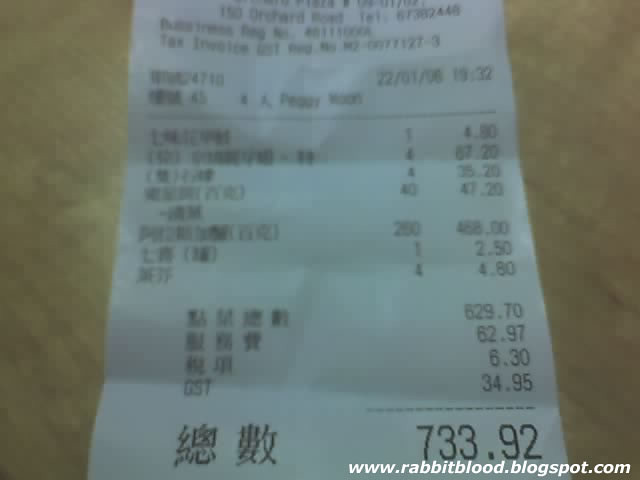A blurry image of a store receipt is displayed prominently against a light wooden background. The focal point is the receipt, which is printed in black font and is difficult to read due to the blurriness. The total amount on the receipt, $733.92, is visible in large black numbers. The receipt lists seven products, though the specific items are not discernible. The receipt also contains a mix of English and oriental writing, particularly noted at the bottom. In the lower left-hand corner of the image, the URL "www.rabbitblood.blogspot.com" is printed in white font twice.